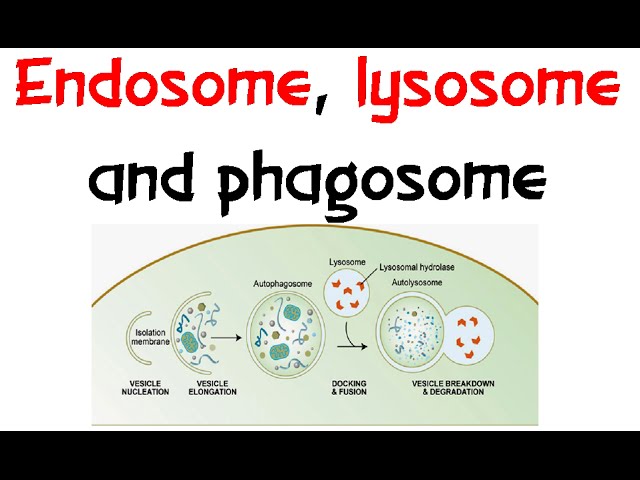The image depicts a detailed scientific diagram explaining various cellular processes on a white background with thick black bars at the top and bottom, resembling a slide from a PowerPoint presentation or a science textbook poster. At the top, red text reads "endosome, lysosome" and black text continues with "phagosome." The central illustration features a sequence within a green semicircle with a yellow trim. Inside the semicircle, the processes start with "isolation membrane" and continue through "vesicle nucleation" and "vesicle elongation." These stages are represented by scientific symbols and arrows pointing to their descriptions.

The diagram then evolves into a full green circle labeled "autophagosome," which is filled with additional scientific symbols. This circle connects to a white circle at the top right marked "lysosome," depicted with red arrow symbols and labeled "lysosomal hydrolase autolysosome." An arrow signifies the "docking and fusion" process that leads to another semicircle. This final stage is captioned "vesicle breakdown and degradation," incorporating more scientific symbols. The right section shows the lysosome combining with the vesicle, illustrating the final degradation phase, thus providing a comprehensive visualization of cellular degradation pathways.